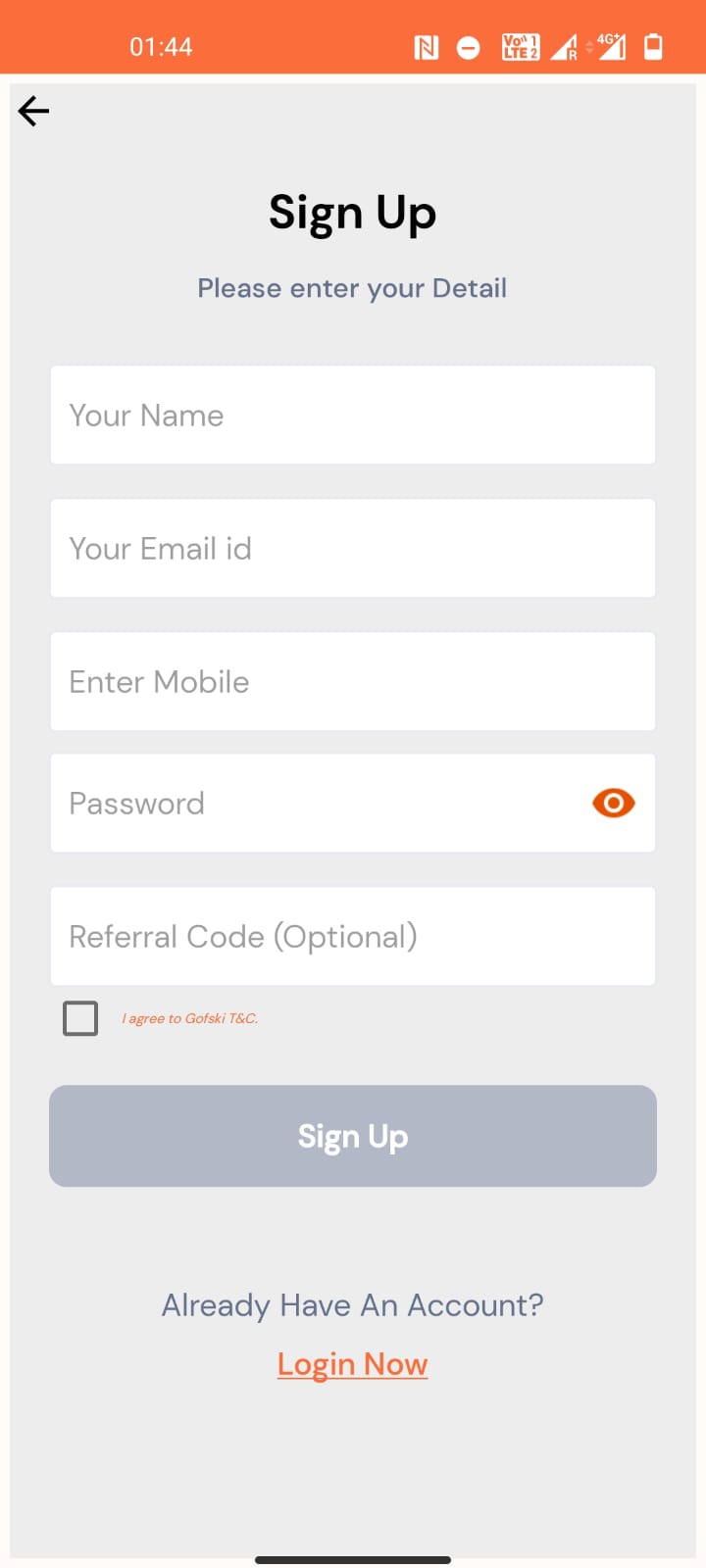A screenshot taken from a smartphone captures a sign-up page within an app. The device’s status bar, encapsulated in an orange shade, stretches across the top, displaying a timestamp of 1:44 on the left side and indicators for battery percentage, Wi-Fi signal strength, and open apps on the right. The main interface boasts a gentle bluish-purple background. Centrally positioned, bold black text reads "Sign Up," followed by a prompt in a slightly darker hue instructing users to "Please enter your details." 

This prompt is followed by five rectangular input fields for the user’s name, email ID, mobile number, password, and an optional referral code. Below these fields lies a checkbox with a light blue background, likely meant to confirm agreement to the terms and conditions, though the complete text isn't fully captured. A black rectangle beneath houses a similarly hued background label, "Sign Up," in white text. Further down, a message inquires if the user "Already have an account," offering an underlined link in orange font that urges, "Log in now."